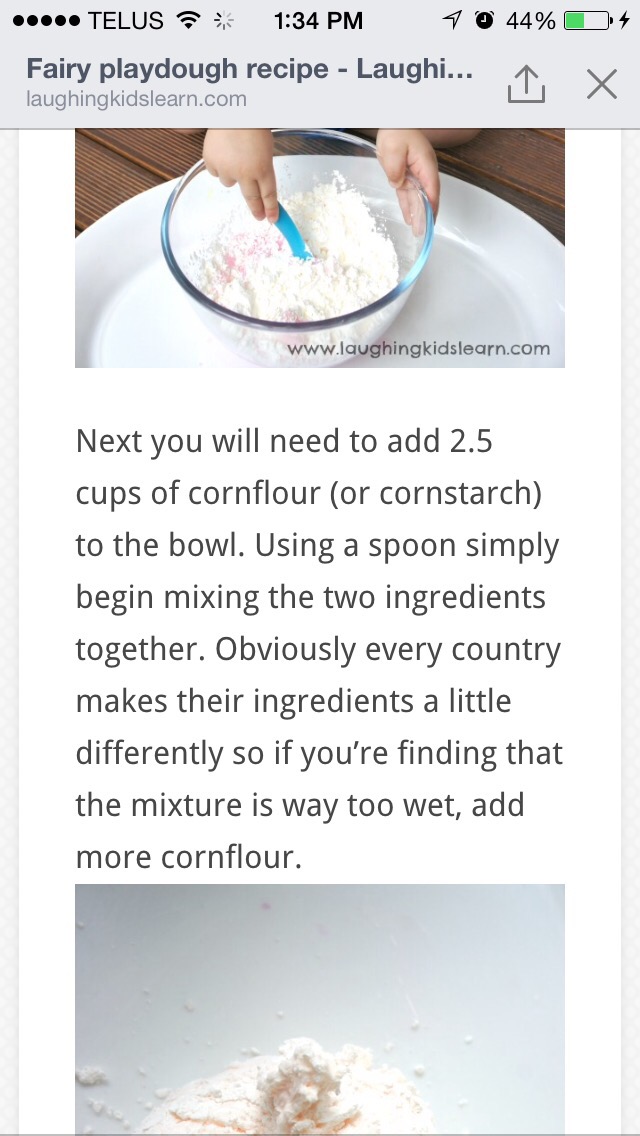The screen capture from a cellphone depicts an indoor setting featuring a detailed recipe for making play-doh from LaughingKidsLearn.com, taken at 1:34 PM with Telus network. The upper part of the image shows typical phone status indicators such as battery level, network connection, and time. The main content displays a white person, presumably a child, stirring a mixture of corn starch in a clear bowl with a blue spoon, placed on a white dish on a brown table. The visual text informs users to add 2.5 cups of corn flour or corn starch to the bowl, highlighting that ingredient measurements may differ by country. If the mixture turns out too wet, additional corn flour is recommended. The lower part of the image includes another photo, likely a close-up, showing corn starch. The website URL, LaughingKidsLearn.com, is also visible in portions of the image, providing a source for the recipe.